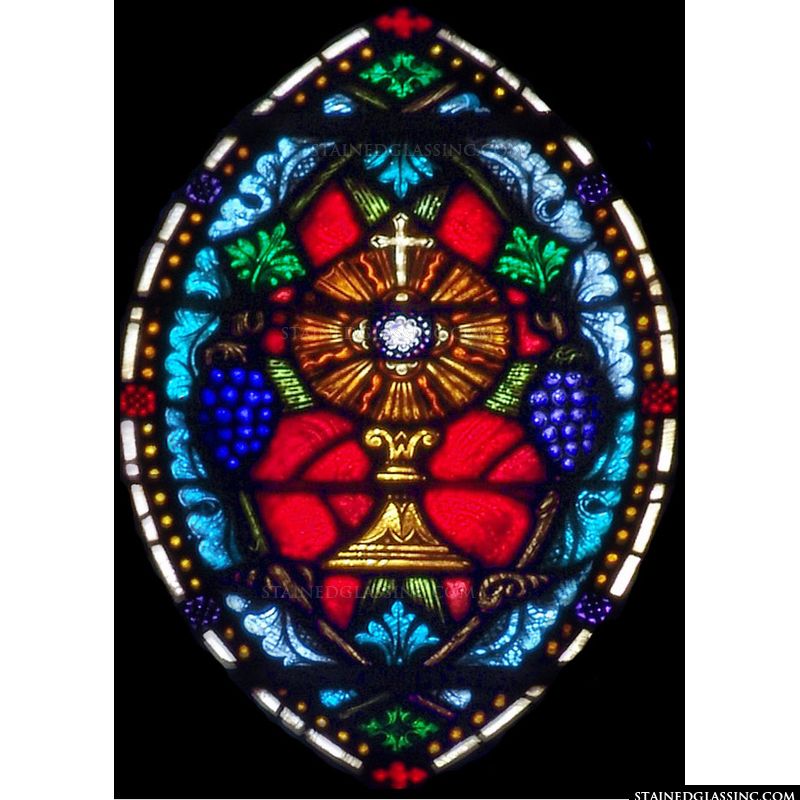This image depicts a vibrant stained glass window with an intricate and colorful design, set against a black background. The window features an oval shape framed by black borders adorned with yellow dots. At each corner of the oval, there are vivid red roses. Within this larger oval lies another oval, accented by bunches of grapes on either side. The central focus is a round circle with a brown border, crowned by a cross, resembling a chalice or candle holder with a glowing white center that resembles a gem. This centerpiece is flanked by red, heart-like areas. Encircling the entire design is a frame that appears whitish and curves elegantly. The stained glass displays a rich palette of colors, including blues, reds, golds, and purples, adding to its ornate appearance. The bottom right corner of the image bears the inscription “stainedglasses.com.” The photo might have been taken through a second barrier, giving it a slightly blurry quality, yet the detailed and colorful design remains strikingly evident.